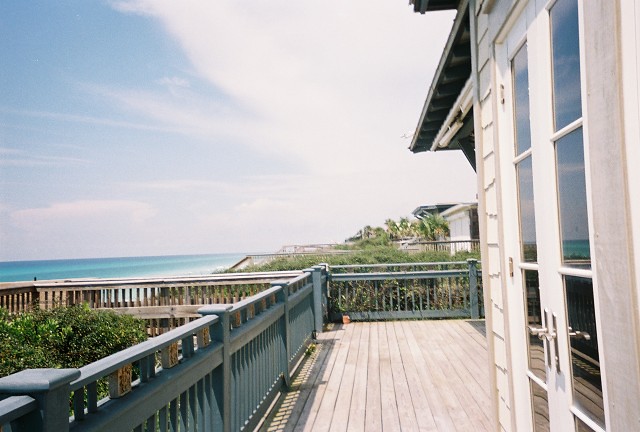The image depicts a scenic view from a beach house deck, showcasing a tranquil seaside atmosphere. To the left, a turquoise blue ocean stretches beneath a mostly blue sky dotted with white, wispy clouds. The beach, adorned with various shrubs and bushes, lies between the water and the row of waterfront houses aligning the coast to the right. 

The foreground features a spacious deck made of grayish-brown wooden planks extending in an L-shape towards the beach. This deck is bordered by a distinct matted teal blue railing with wooden columns supporting a horizontal board. On the far right side, partially visible, are French doors with reflective glass panes, framed by white wood, inviting glimpses of the sky's reflection within. The deck's wooden structure and surrounding shrubbery fuse with the serene coastal landscape, capturing the serene beauty of a tropical beachfront setting.